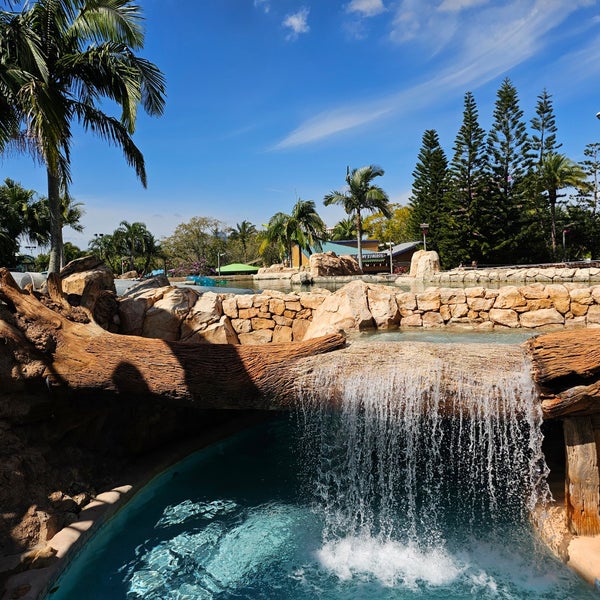This digital photograph captures a serene, man-made waterfall scene at a resort. In the foreground, a clear blue pool of water is fed by a stream cascading over a large wooden log, flanked by a stone wall that appears deliberately constructed. To either side of the pool, rocks and additional stone structures create an organized, almost natural appearance. A variety of trees, including palms and evergreens, populate the background, enhancing the tranquil setting. The bright blue sky, streaked with wispy white clouds, adds to the picturesque ambiance. To the far left, near the log, stand a few palm trees, adding a tropical touch. In the distance, colorful housing with triangular but flat roofing, painted in hues of green and blue, peeks through the foliage. Illuminated by sunlight, the entire scene emits a warm and inviting glow, although the absence of people lends it a somewhat static and almost frozen quality.